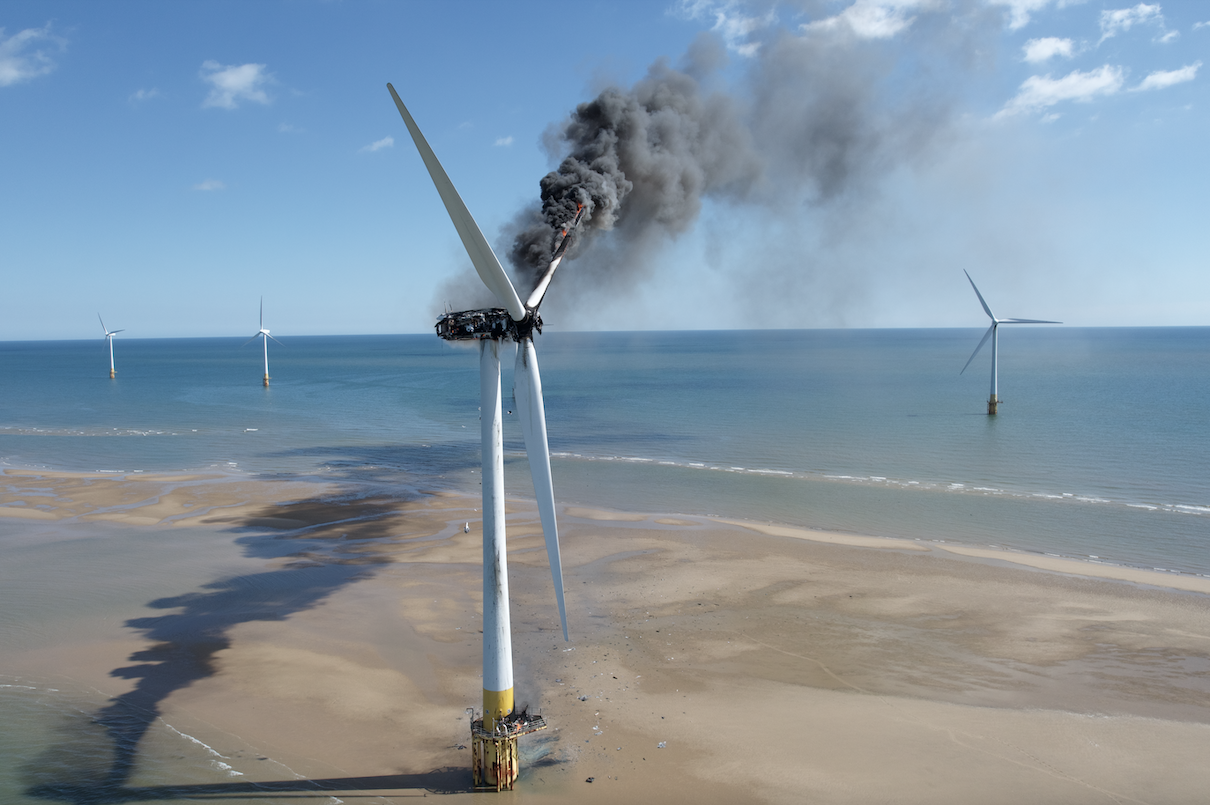This is a detailed photograph of an electric-generating windmill engulfed in flames. The windmill, designed to harness energy from the wind, stands attached to a large, thick white pole, which is painted yellow at its base. Surrounded by sand and water, it clearly marks it as a shore windmill. The image showcases other similar windmills in the background, situated in the ocean. The windmill in focus has its top blackened and gutted by fire, with large gray and black smoke clouds billowing from the engine and the damaged blade. The windmill features three blades: two remain white, while the third is charred and ablaze. Additional flames are visible on the platform at the base of the structure. The sky is mostly clear with patches of clouds, accentuating the dramatic scene.